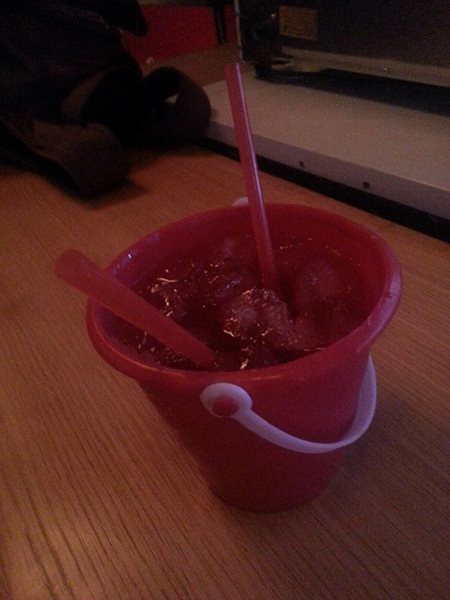In the photograph, a small red toy bucket, roughly the size of a large cup, features prominently. The bucket, typically reminiscent of children's beach toys, has a white plastic handle that hangs down its sides, curving slightly. This bucket has been whimsically repurposed as a drinking vessel, filled with ice and a red or dark pink liquid—potentially reflecting the bucket's color. Two red straws protrude in opposite directions from the top of the bucket. The scene unfolds on a wooden tabletop or desktop, creating a rustic backdrop. In the background, there’s a hint of an upside-down black cat, adding a playful touch to the image. The unconventional drink setup, with its icy refreshment and unusual container, stands out against the wooden surface, possibly part of a workstation.